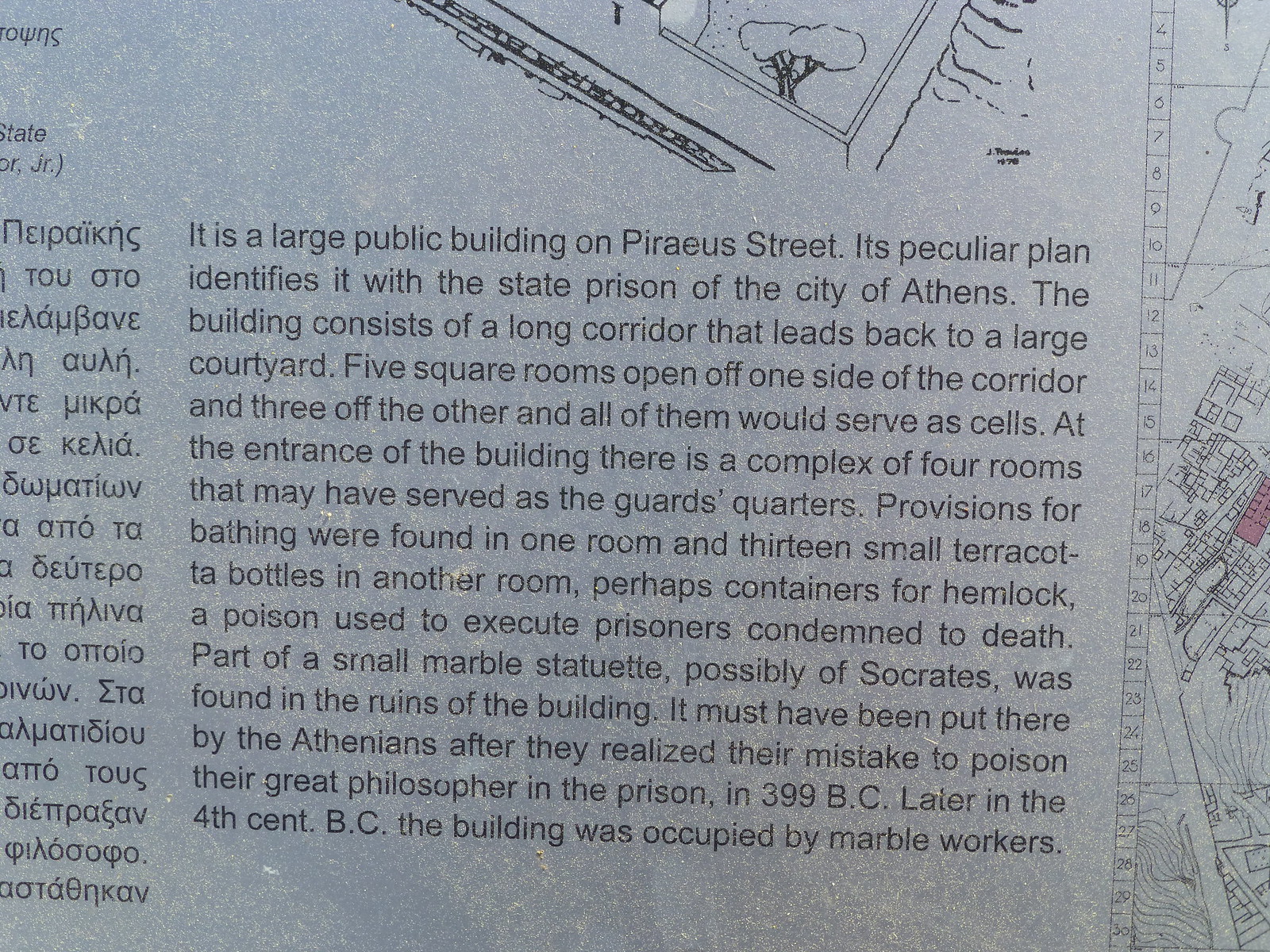The image appears to be a photograph of a textured, gray page from a book, featuring descriptive text etched in black. The page has a mottled blue distortion, adding to its aged look. The top part of the page includes a line drawing depicting a corner of a courtyard featuring a tree and walls. A bit of a column on the left-hand side shows writing in Greek. The central part contains detailed information about a historical building, likely the state prison of Athens, located on Piraeus Street. The building's floor plan reveals a long corridor leading to a large courtyard, flanked by five square rooms on one side and three on the other, all serving as cells. At the entrance, a complex of four rooms may have been used as guards' quarters, with provisions for bathing found in one room and 13 small terracotta bottles—possibly for hemlock, a poison for executing condemned prisoners—discovered in another. Notably, part of a small marble statuette, potentially of Socrates, was found among the ruins, hinting at the Athenians' remorse for poisoning the philosopher in 399 BC. During the 4th century BC, marble workers occupied the building.